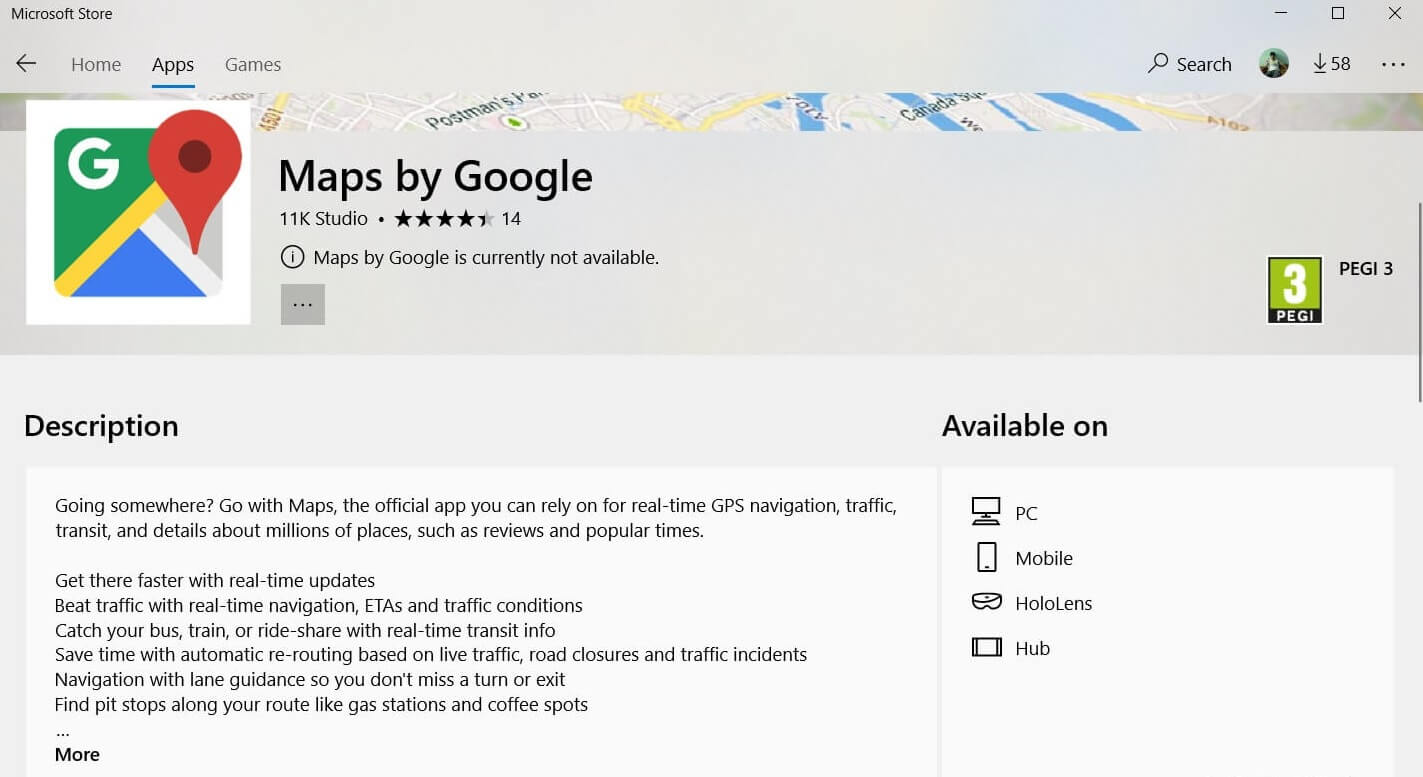This detailed caption describes a screenshot of the Microsoft Store interface that is focused on the "Apps" section.

---

In this screenshot of the Microsoft Store, we are presented with the main navigation tabs at the top: Home, Apps, and Games. The "Apps" tab is currently selected and underlined. A thin promotional banner spreads across the entire width of the top, featuring a tilted view of a Google Maps interface. Below this banner, the search bar, user profile icon, and a download icon indicating 58 current downloads are visible.

Beneath the main navigation, there's a prominent white overlay partially covering the banner on the left. This overlay features the Google Maps icon. To the right of the icon is the app title "Maps by Google," credited to "11K Studio," and rated at four and a half stars out of fourteen total ratings. Notably, "Maps by Google is currently unavailable" is displayed, indicating the app cannot be downloaded at the moment.

The descriptive section for Google Maps reads: "Going somewhere? Go with Maps, the official app you can rely on for real-time GPS navigation, traffic, transit, and details about millions of places such as reviews and local conditions. Get there faster with real-time updates including speed, traffic conditions, ETAs, and traffic information. Catch your bus, train, or rideshare with real-time transit info. Save time with automatic rerouting based on live traffic, road closures, and traffic incidents. Navigate with lane guidance to avoid missing turns or exits. Find pit stops along your route like gas stations and coffee spots. The app is available on PC, mobile, HoloLens, and Hub, with icons representing these platforms displayed next to the description."

---

This caption provides a comprehensive description of the visual elements and text within the Microsoft Store screenshot.